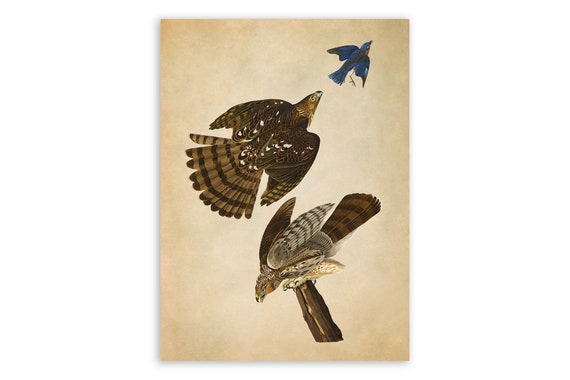This piece of art depicts a dramatic aerial scene with three birds against a muted, beige-grey background. In the top right corner, a vibrant blue bird, possibly a blue jay or robin, ascends with partially obscured red markings on its chest. Below it, a brown hawk with dark and light horizontal striping on its fully extended wings and tail seems to be in pursuit. The hawk’s body features distinctive white speckles. In the bottom right, another bird, which appears to be a lighter-colored hawk or eagle, is perched atop a tree branch. This perched bird may have captured a smaller white bird or animal beneath it, adding a possible theme of hunting to the artwork. The absence of a signature and the dynamic composition give this painting a raw and engaging feel.